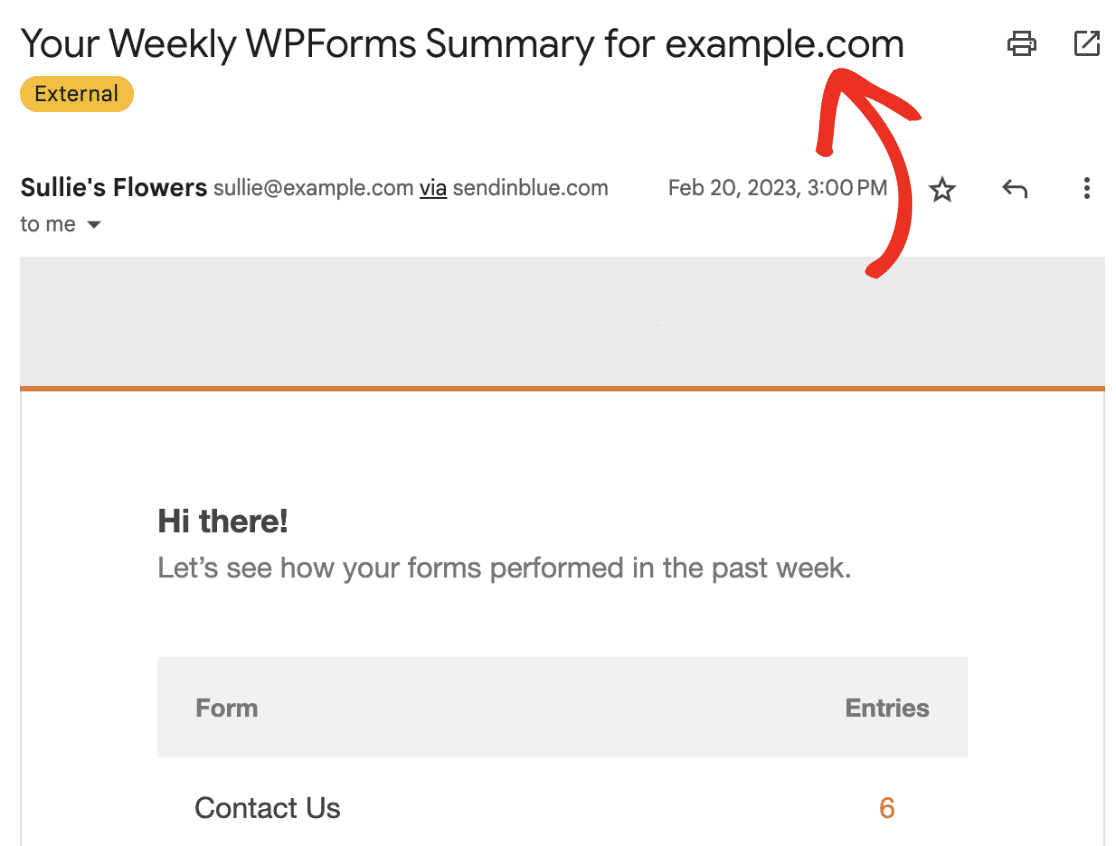Screenshot of a Work Management Tool Generating Weekly Email Summaries

This image captures a screenshot from what appears to be a work management tool focused on generating email summaries. The page features a header in bold black text on a white background that reads, "Your Weekly WP Forms Summary," indicating that this may be a training template for WP Forms users.

Below the heading, there's a gold button labeled "External" positioned in the upper left corner. Beneath that, there is a bolded subheading, "Sully's Flowers," followed by the email address "sully@example.com" via "sendinblue.com," suggesting that this email is facilitated through the Sendinblue platform.

Further down, the email content starts with a greeting, "Hi there, let's see how your forms performed in the past week." This is followed by a section highlighting form entries. A blue banner on the left, labeled "Form," is paired with the number of entries on the right. Specifically, it mentions a "Contact" form with 6 entries.

The overall layout and content suggest that this screenshot serves as a tutorial for navigating and understanding the WP Forms summary, likely aimed at users of the tool.